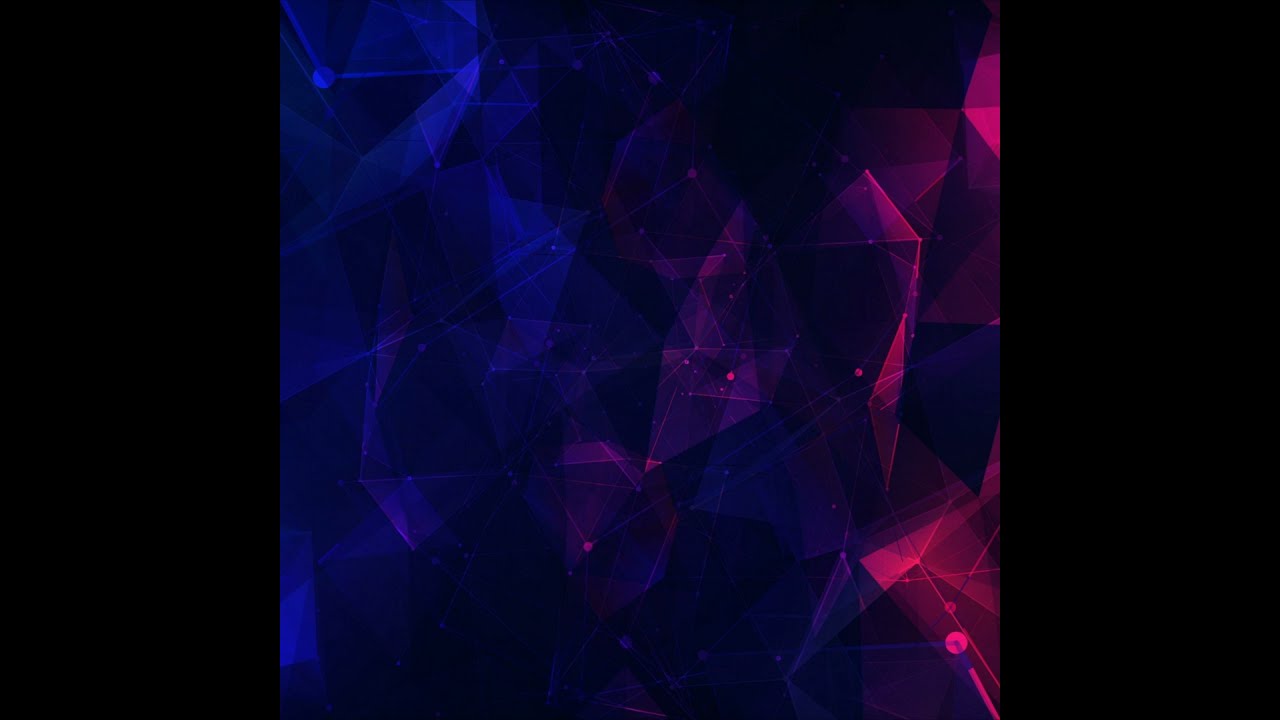This image showcases a striking 3D geometric design, ideal for use as computer or laptop wallpaper. The central artwork is framed by black rectangular borders on both sides, adding depth. The composition consists predominantly of transparent, interconnected triangles and rectangles, creating a layered, shard-like effect. The color palette transitions fluidly across the image: starting with deep blue hues on the left, shifting to darker blues and purples in the center, and culminating in vibrant pinks on the right. Additionally, the design features white lines with small dots that connect various shapes, enhancing its complexity and abstract nature. Set against a mostly black background, the overall aesthetic is both futuristic and modern, characterized by its intricate geometric patterns and vivid gradients.